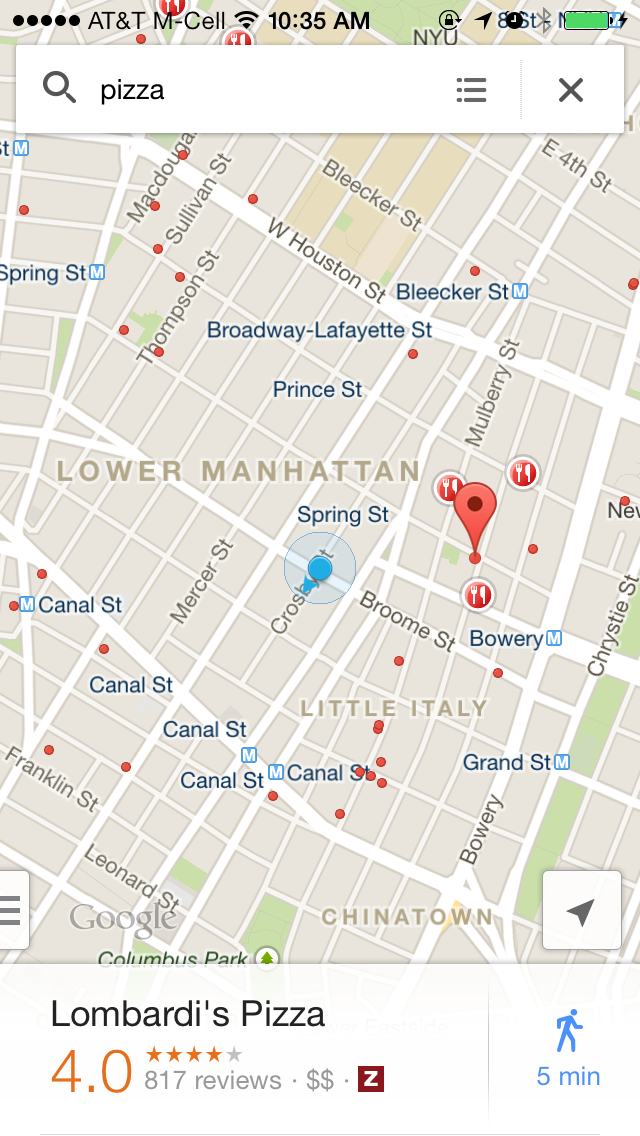A Google Maps search for Lombardi's Pizza in Lower Manhattan is displayed on an AT&T phone. The interface shows the user's current location as a blue dot and Lombardi's Pizza as a red location icon. The map indicates it is about a five-minute walk, suggesting the user is roughly three or four blocks away. Streets surrounding the routes are clearly labeled. Additionally, Lombardi's Pizza is highlighted with a rating of 4.0 based on 817 reviews. The search term "pizza" appears at the top of the search screen. This visual does not include the detailed step-by-step directions but focuses on the initial search results and route overview.